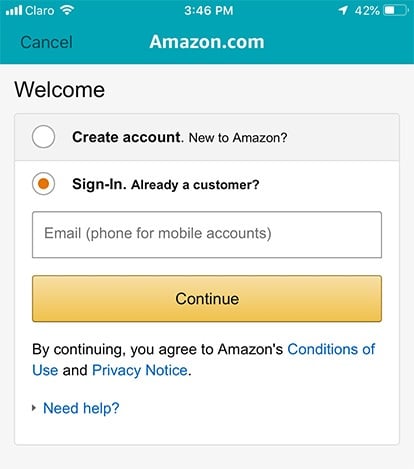The image depicts a screenshot from an older model iPhone with Claro as the service provider. The status bar indicates that the time is 3:46 PM, with the battery life at 42% and the Wi-Fi indicator showing connectivity. The screenshot captures an Amazon.com login page, characterized by its outdated design reminiscent of the 2015-2018 era. The page welcomes users with options to either create a new account or sign in if they are already customers. The "Already a customer? Sign in" option is selected, revealing a field for entering an email or phone number for mobile accounts. Below this, there's a "Continue" button, with a note that proceeding implies agreement to Amazon's conditions of use and privacy notice, both of which are clickable for further reading. Additionally, there is a "Need help?" link suggesting a dropdown menu for assistance. The overall resolution of the screenshot is notably low, further hinting at the older technology used to capture this image.